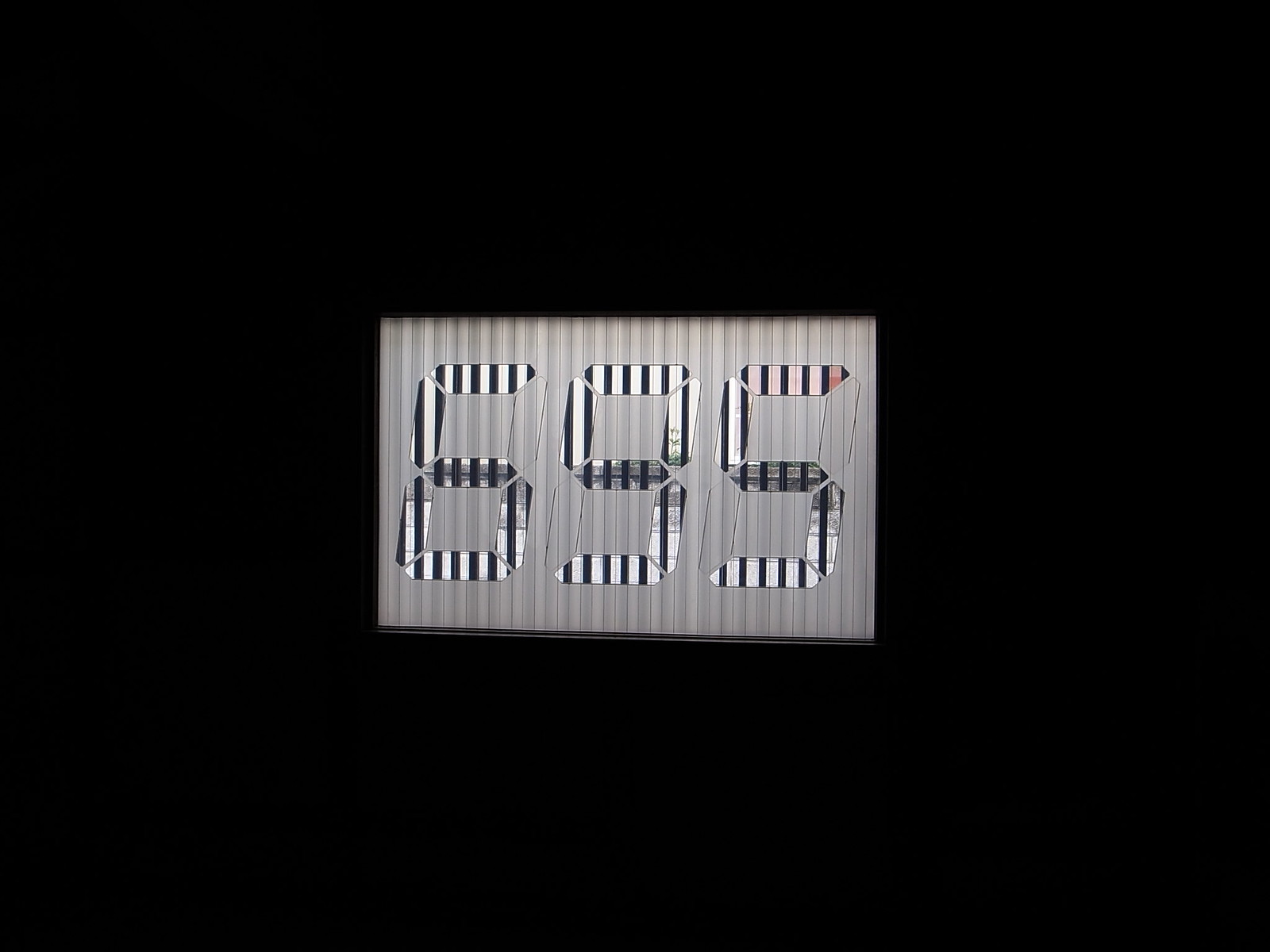This rectangular image features a solid black background, providing a stark contrast to a prominent central photograph. At the heart of this image is what appears to be a segment of a digital display, potentially an electronic reading of some sort. The display does not resemble a clock due to the absence of a colon separating the numbers. 

Spanning horizontally in the background is a subtle gray stripe, adding a touch of texture to the otherwise monochromatic scene. The numbers themselves are striking with their black and white vertical stripes and display the value "695."

Enhancing the realism of the display, a thin medium-gray border runs along the bottom edge, imparting a slight three-dimensional effect. Notably, the black background is perfectly flat without any shadowing, emphasizing the clarity and minimalism of the composition.